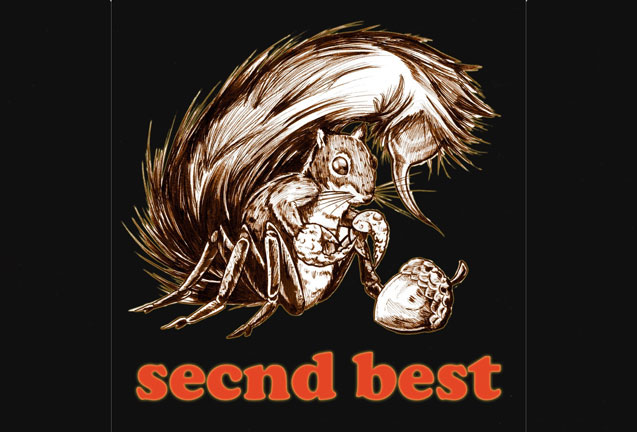The image is a detailed and somewhat eerie illustration set against a predominantly black background. Central to the composition is a chimera-like figure of a squirrel with insect and arachnid features, prominently drawn in a pencil sketch style. This bizarre creature has six elongated beetle-like legs, lobster-like pincers for hands, and a large bushy tail that ends in a scorpion's stinger. The squirrel appears to be fixated on a large acorn placed in front of it. Surrounding the creature, at the bottom of the image, are the words "Second Best" spelled out as "S-E-C-N-D Best" in bold red letters. A distinct, thin light gray border frames the central section of the artwork, enhancing the visual separation from the dark background. The primary colors in the image are black, red, and white, creating a stark and unsettling contrast.